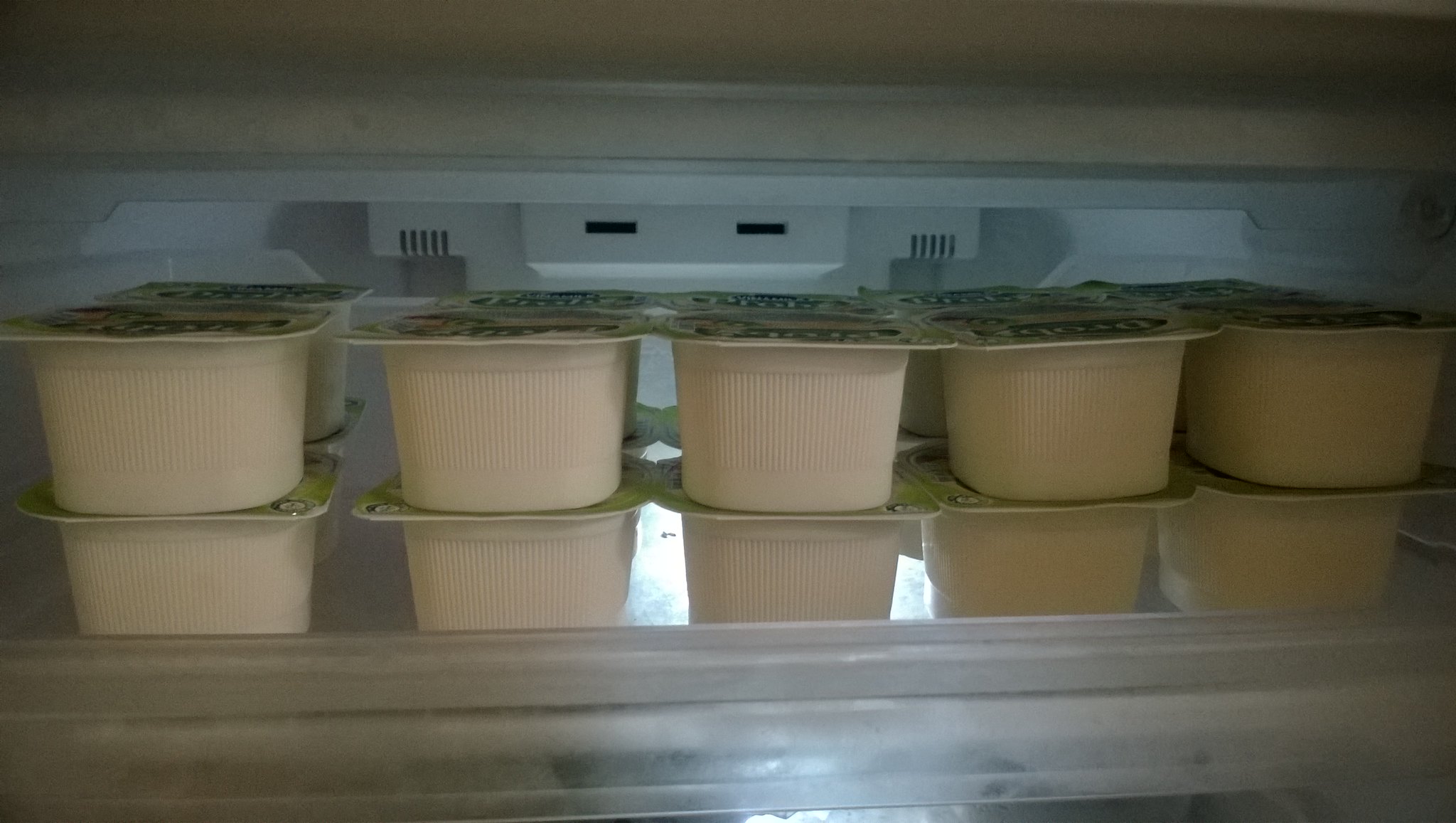The image shows a close-up view of a shelf within what appears to be the top section of either a refrigerator or a freezer, characterized by its white plastic interior. On this shelf, there are two rows of small, white plastic cups with foil lids, neatly stacked in two tiers, totaling twenty cups altogether. The cups are organized five per row, with two rows in the front and two rows directly behind. Although the exact contents of these cups are unclear due to the oblique angle and the indistinct print on the lids, they are likely single-serving yogurt or pudding cups. The shelf appears to be made of glass, as there are reflections visible, and there are tiny ventilation ducts or rectangular holes at the back, reinforcing the refrigeration context. The contents in the cups, or perhaps the cups themselves, look white, suggesting a creamy, dairy-based product.